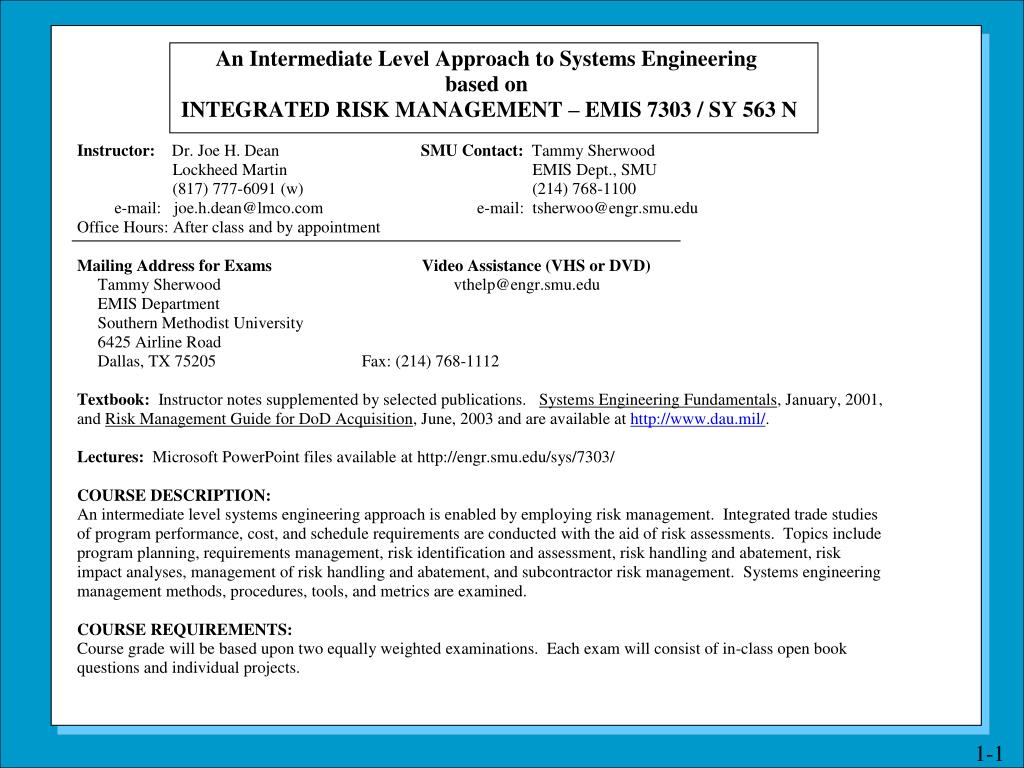Here’s a cleaned-up and detailed caption for the described image:

---

At the top of the image, within a rectangular border, the title reads "An Intermediate Level Approach to Systems Engineering Based On" followed by the text in uppercase "INTEGRATED RISK MANAGEMENT" and the course code "EMIS 7303 - SY563N".

Directly beneath this title, the text is presented in two columns. On the left side, in black font, it states "Instructor: Dr. Joe H. Dean". On the right side, it reads “SMU Contact: Tammy Shepard”.

A horizontal line separates these sections from the next area below, which contains information in two parts. The left side mentions "Mailing Address for Exams" and the right side specifies "Video Assistance (VHS or DVD)".

The following section lists "Textbook" with "Lectures" written underneath. To the right of this, there is a note that "Microsoft PowerPoint Files Available".

Further down, the image includes a "Course Description" area, which provides an overview of the course content and objectives.

The final section, emphasized in bold black print, is labeled "Course Requirements". It explains that the course grade will be based on two equally weighted examinations. Each exam entails in-class, open-book questions, and individual projects. This is the concluding piece of information in the image.